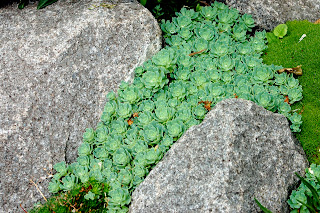This photograph, taken outdoors, captures a close-up view of a serene garden scene. Dominating the left side of the image is a large gray, rough-edged boulder, complemented by a smaller, similarly rugged stone in the bottom right corner. Nestled between these stones is a lush cluster of round petal-like succulent plants, likely stonecrop or miniature cabbages, their vibrant light green leaves spreading abundantly across the space. A smaller patch of green plants coexists with the succulents in the bottom left. Just above the stone in the bottom right, a patch of green moss adds a soft contrast. Additionally, another rock appears partially in the top right, blending into the natural mosaic. The overall scene is a peaceful display of nature's resilience and beauty, with a grassy patch to the right and the succulents' bright greenery highlighting the tranquil garden setting.